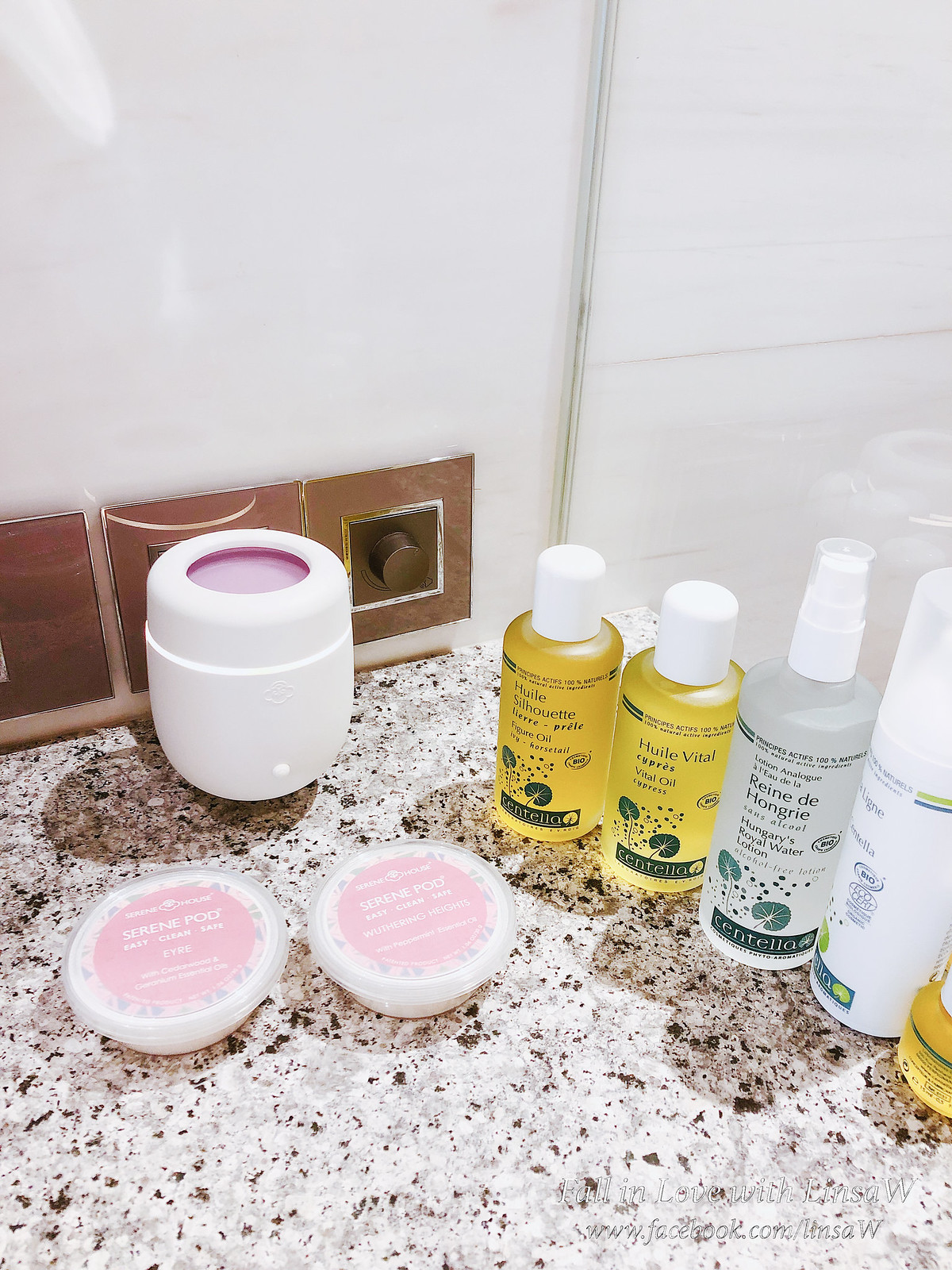The photograph showcases an array of skincare products neatly arranged in what appears to be a bathroom setting. The background features a glossy, white-tiled wall adorned with three brown square tiles. On the rightmost tile, a turn dial knob is visible, though its function remains unclear—it could be a light dimmer or some other control device.

Front and center stands a white, rounded plastic device with a purple opening at its top, possibly a mister. In front of this device are two circular plastic containers inscribed with "Serene Pod Easy Clean Safe." The container on the left is labeled "EYRE," while the one on the right reads "Wuthering Heights."

To the right of these containers are two bottles filled with a yellow-tinted oil, each capped with a white lid. The labels on these bottles read "Centella HUILE Silhouette Figure Oil" and "Centella HUILE Vital Cypress Vital Oil Cypress Centella."

Next to these bottles is a clear container labeled "Lotion Analog Reindehungere Hungarian's Royal Water Centella." Adjacent to it lies a white bottle with a clear cap turned sideways, though its label is not entirely visible.

All of these items rest atop a white and brown speckled marble countertop, adding to the aesthetic appeal of the arrangement.